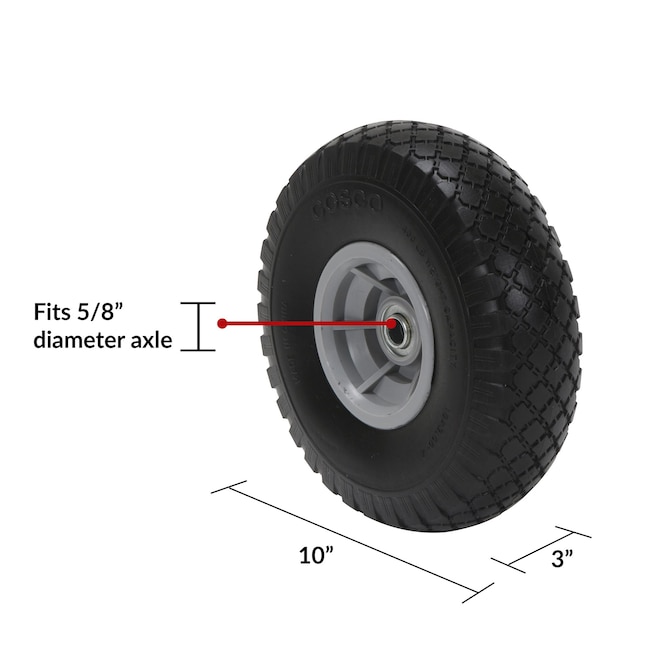This image showcases a black tire branded "COSCO" (C-O-S-C-O) with distinctive tread, appearing brand new against a plain white background. The tire features a detailed hub in the center, which is a dull, silver-gray metal and includes a central hole. Surrounding this hole is a measurement label that indicates the tire fits a 5/8-inch diameter axle. There are several colored lines around the tire to indicate dimensions: a red line leads from the center of the hub to the outer edge, highlighting the axle fitment, while other lines measure the tire's dimensions. The length of the tire is marked as 10 inches, and the breadth (or width) is 3 inches. This meticulously depicted tire is clearly labeled and measured for detailed specification.